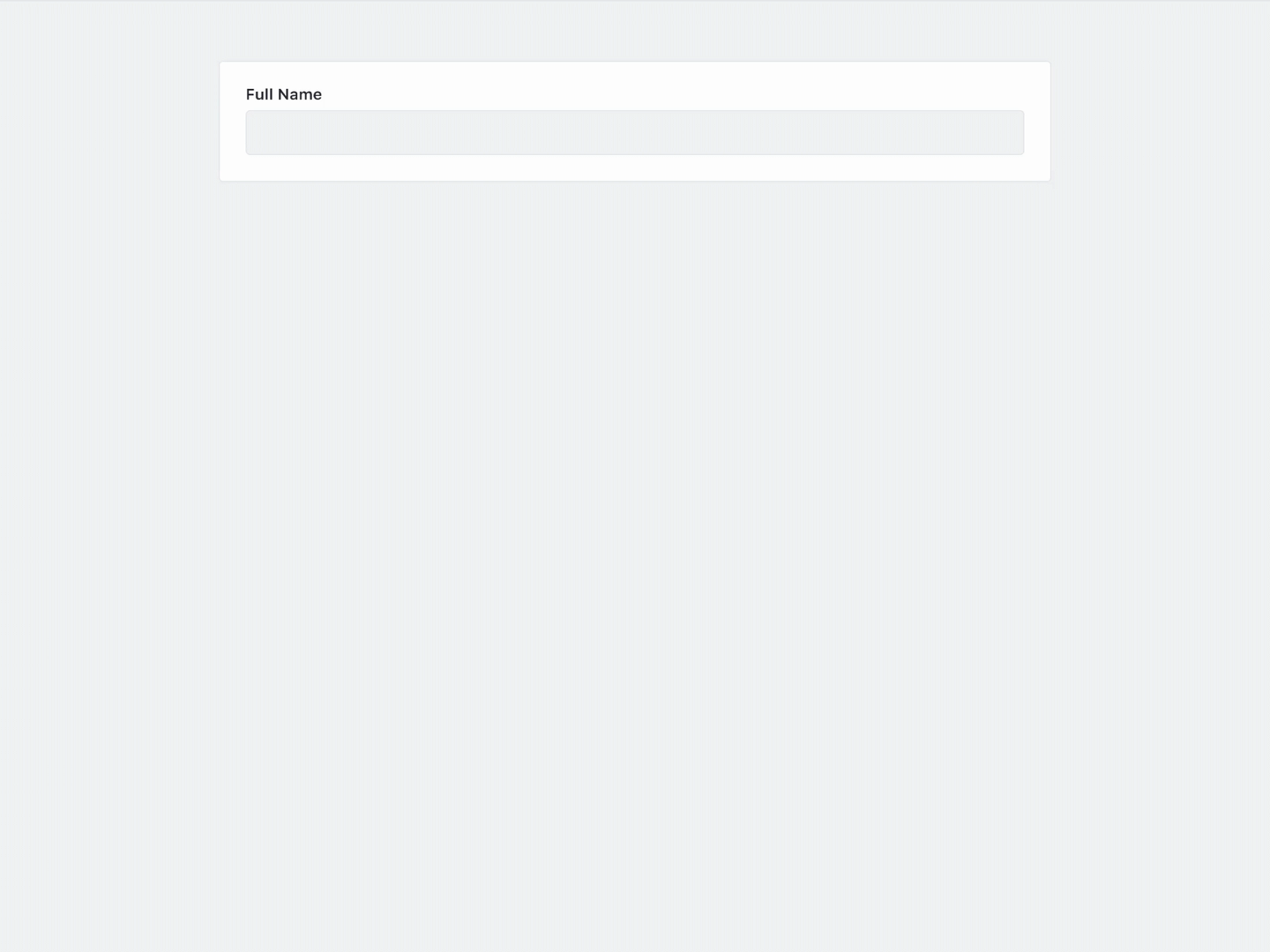The image features a very light gray square background, which occupies the entirety of the canvas. Positioned within the top fourth of the square is a centered white rectangle. Inside this white rectangle, there is a full name written in black text. Beneath the white rectangle is another rectangle, which is the same shade of light gray as the background, creating a subtle, almost imperceptible effect. This gray rectangle spans the same width as the white rectangle, leaving white margins on the top, left, and right sides. The bottom part of the gray square background, accounting for approximately two-thirds of the overall height, is entirely empty, contributing to the spacious and minimalist aesthetic of the design. The overall color palette consists of light gray, white, and black tones. This image appears to be an unfinished design or a placeholder, potentially intended for use in a web form or a digital interface where elements might be added later.